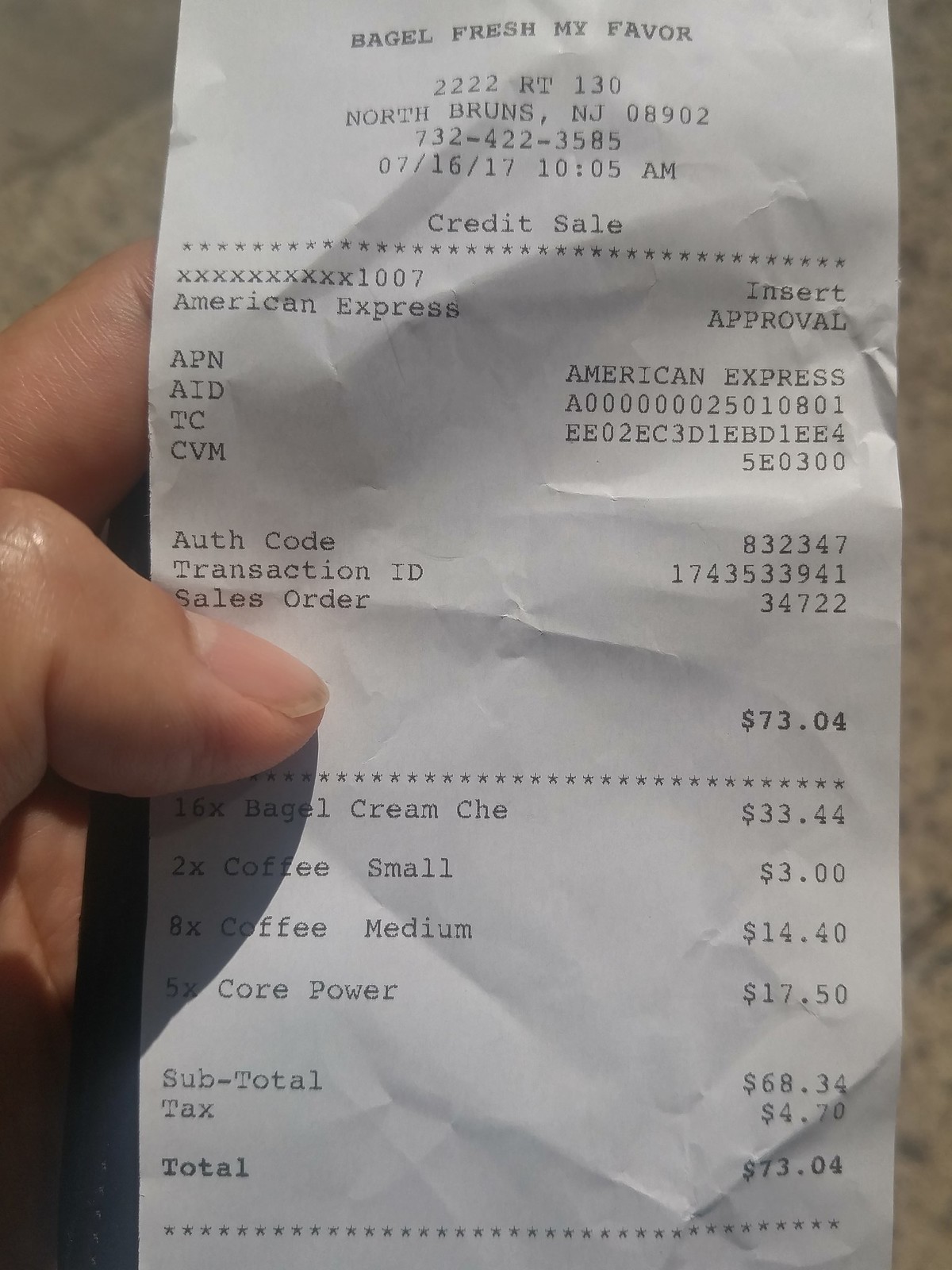The color photograph features a close-up view of a person's thumb holding a white receipt. The receipt is from Bagel Fresh My Favor, located at 2222 Route 130, North Brunswick, New Jersey, 08902. The store's contact number is printed as 732-422-3585. The receipt is dated July 16th, 2017, and timestamped at 10:05 AM. It reflects a credit sale transaction made using an American Express card.

Key details of the receipt include:
- Store and Transaction Information: 
   - A credit sale using American Express with insert approval, APN, AID, TC, CVM, and approval code details. 
   - Transaction ID is 1743533941 and Sales Order is 34722.
- Purchased Items:
   - 16 Bagels with Cream Cheese: $33.44
   - 2 Small Coffees: $3.00
   - 8 Medium Coffees: $14.40
   - 5 Core Powers: $17.50
- Financial Summary:
   - Subtotal: $68.34
   - Tax: $4.70
   - Total: $73.04

The image prominently highlights the detailed text and numerical components on the receipt, capturing the multitude of items purchased and the total amount spent.